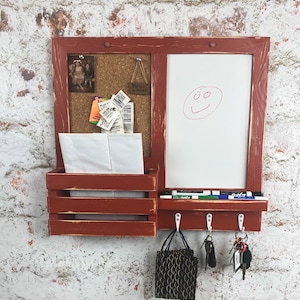This detailed photograph depicts a compact, red wooden hall organizer mounted on a dirty rock wall. Designed to assist in storing valuable items and making quick notes, the organizer has several distinct features. On the left-hand side, there is a cork board framed in red wood, adorned with a variety of items: a picture at the top, small labels, and receipts pinned in the center, and a string hanging from a hook. Below the cork board is a small basket that holds miscellaneous papers, likely mail. The right-hand side features a whiteboard, on which a red smiley face has been drawn. Below the whiteboard, there is a ledge lined with dry erase markers. Underneath this ledge, there are three hooks; from left to right, they hold a bag, a set of keys possibly with a fob, and a larger set of keys attached to a keychain with multiple items. Through its design and arrangement, the hall organizer serves as an efficient tool for keeping important items and notes in one accessible place.